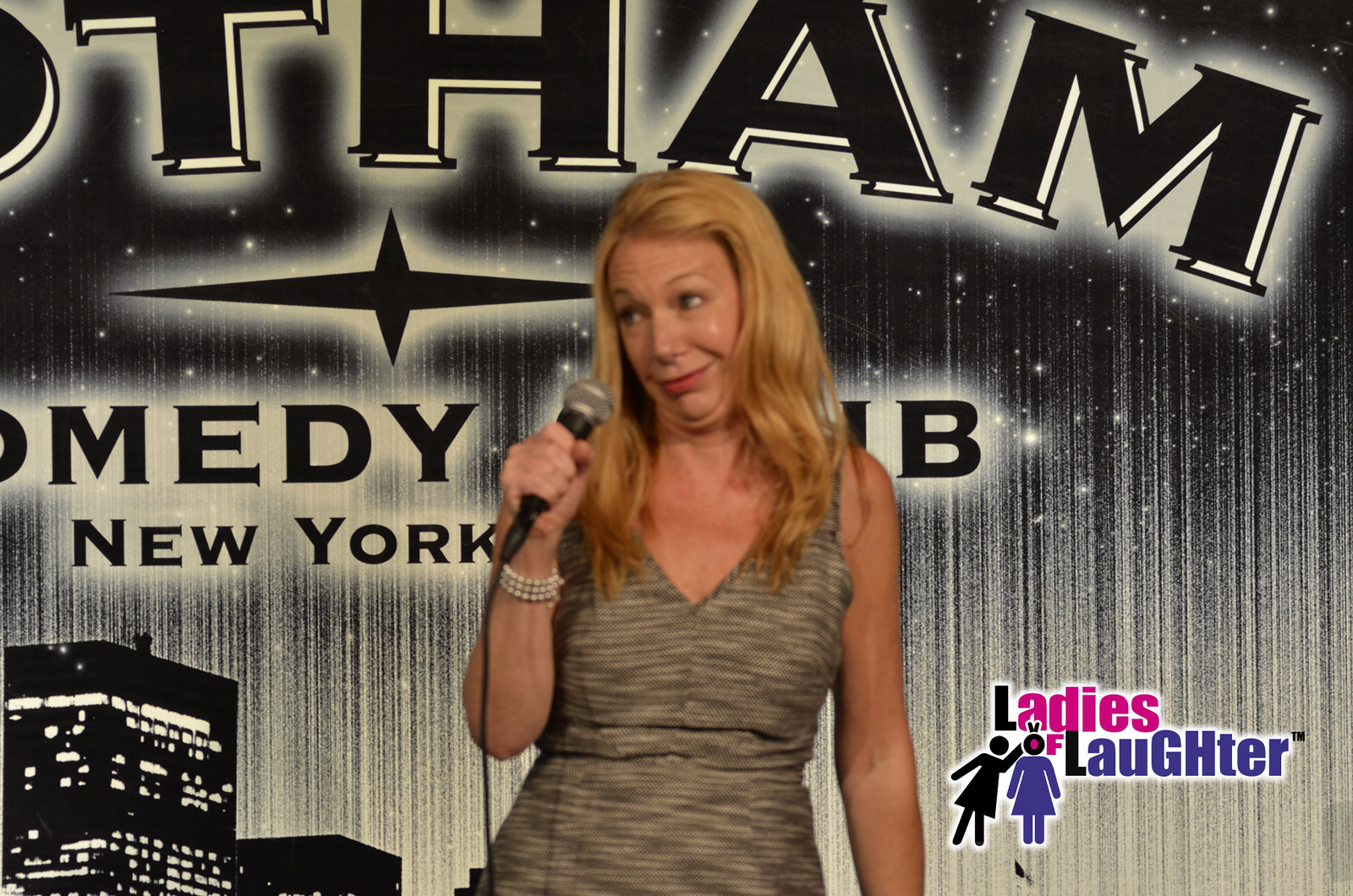The image captures a moment at a comedy event held at the Gotham Comedy Club in New York. Dominating the background is the club's partially visible neon sign, which reads "Gotham Comedy Club New York." The backdrop is supplemented with an impressionistic view of high-rise buildings, hinting at the iconic New York skyline. Center stage is a middle-aged woman, likely in her early 40s, with long, blonde hair and pale skin, who seems to be performing or reacting humorously with a playful, slightly judgmental expression as she glances to her right. She is dressed in a sleeveless, textured gray dress featuring a V-tapered neckline, and accessorizes with a pearl bracelet on her right wrist, which is also holding a microphone, the wire trailing down. The bottom right corner of the image is marked with the logo "Ladies of Laughter," indicating the event's association with this comedy organization.